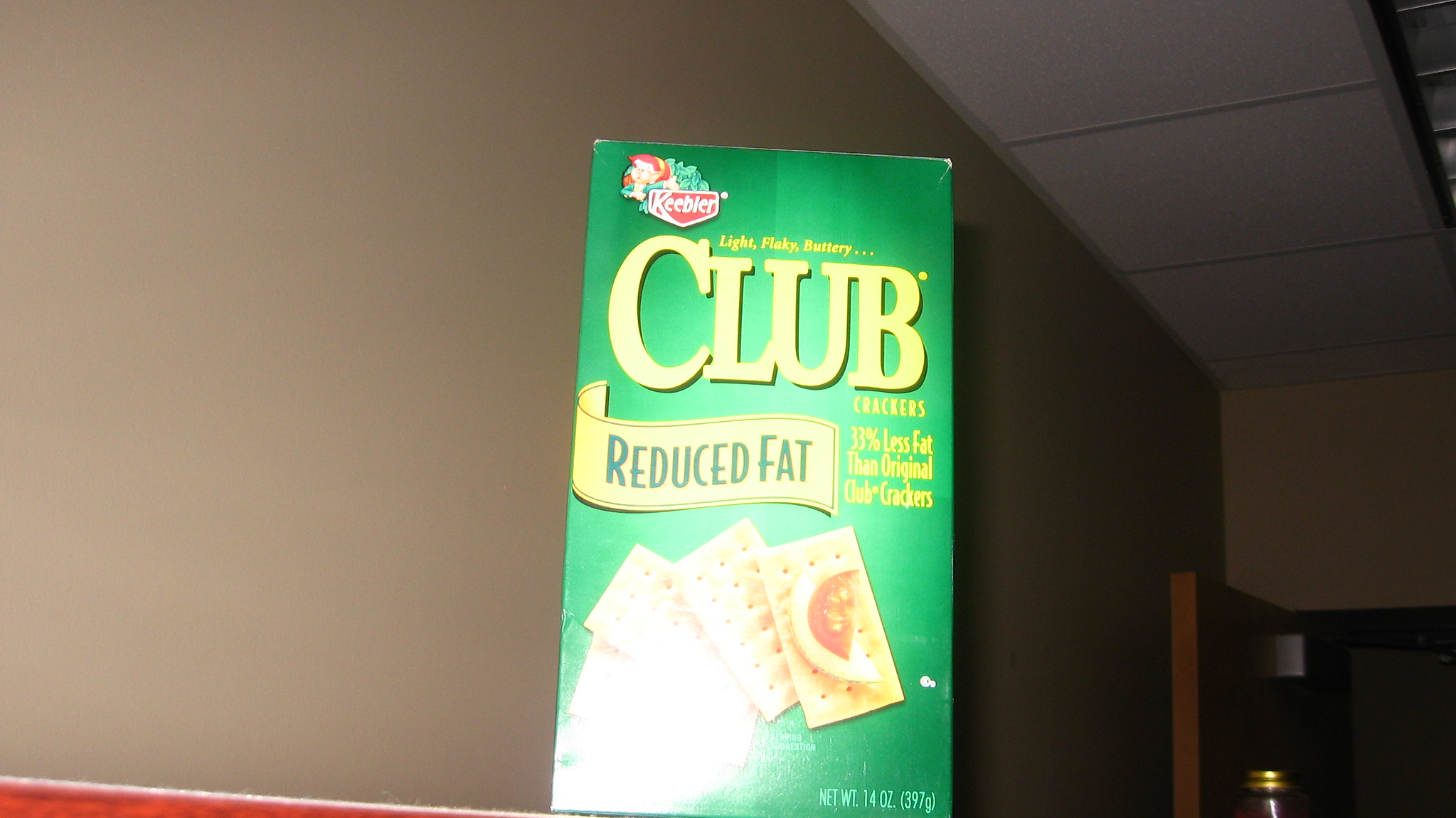In a room with gray walls and a ceiling that resembles an office or school setting, a box of Keebler Club Reduced Fat Crackers is prominently displayed on a table. The box features the Keebler logo with the smiling elf, known as Ernie, positioned in the upper left corner. Below the logo, the word "Club" is boldly printed in yellow against a green background. This particular variety of crackers touts "33% Less Fat than Original Club Crackers". An appetizing image of a cracker topped with a slice of tomato graces the front of the box. A camera flash has slightly obscured the left-hand corner of the box, suggesting the photo was taken with a copious amount of light.